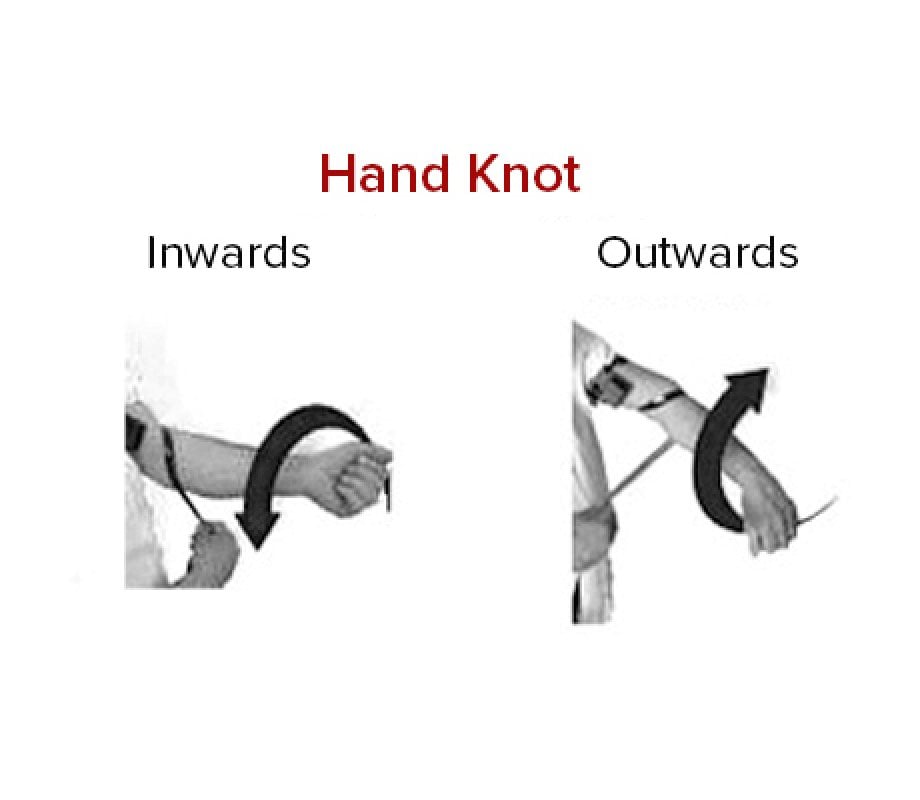The photograph is a detailed instructional guide on how to create a hand knot, prominently titled "Hand Knot" in red letters at the top. The visual is divided into two sections to illustrate the complete process. On the left side, labeled "inwards" in black letters, it depicts a man wearing a short-sleeved white shirt, with his left arm extended outward. An arrow indicates the direction in which a black cord should be wrapped inwards towards the person's body, encircling the upper part of the arm. You can clearly see a part of his torso as he holds the end of the cord underneath his arm with his other hand. On the right side, labeled "outwards," the same individual is shown extending his arm again, but this time an arrow illustrates the cord being looped outwards, away from the body. The step-by-step arrows guide how to rotate the arm to create the outward twist needed to complete the hand knot.